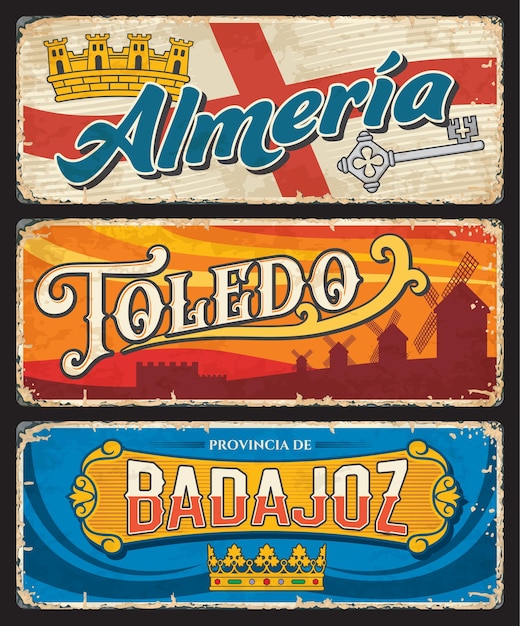This image features a collage of three aged, rectangular advertisements stacked vertically against a black background. The weathered appearance of the pieces suggests age, with rough corners and areas of missing paint, giving them a vintage look.

At the top, the advertisement has an off-white background with a bold, red cross in the center. In blue letters outlined in white, it reads "Almerica" (or "Elmeria"). The upper left corner showcases a yellow, castle-like tower, and the lower right has a silver, skeleton-style key.

The middle advertisement is similar in size and features the text "Toledo" in white on the upper left, accompanied by a yellow swirl beneath it. It predominantly displays four windmills in black silhouette against a striking yellow and orange sky, with a castle faintly visible in the background.

The bottom advertisement, also rectangular, has a blue background and reads "Provincia de Badajoz" in white at the top. Below, there's a gold crown, adding a regal touch to this piece of the collection.

Together, these elements create a cohesive vintage-themed collage, with each advertisement contributing distinct colors and motifs.